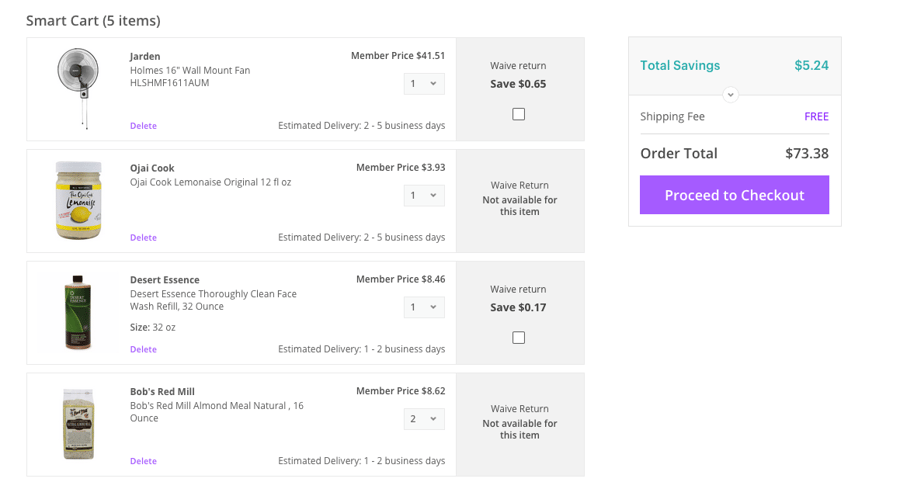This image displays a screenshot from a shopping site. In the upper left corner, it shows a gray text reading "Smart Cart" with a total of five items listed. The items are as follows:

1. **Jarden Holmes 16-Inch Wall Mount Fan**: The fan is priced at $41.51 for members, with a Wave Return savings of $0.65. An image of the fan is provided at the top of the list.
  
2. **Oyaj Cook Lemonaise Original**: This item is a 12-fluid ounce jar of original lemonaise, available at a member price of $3.93. The estimated delivery time for this product is between 2 to 5 business days.

3. **Desert Essence Thoroughly Clean Face Wash Refill**: Offered in a 32-ounce size, this face wash has an estimated delivery time of 1 to 2 business days and is priced at $8.46 for members.

4. **Bob's Red Mill Almond Meal Natural**: This 16-ounce product is listed at a price of $8.62.

The cart summary emphasizes the convenience and savings available to members, detailing each product with its specific price, size, and estimated delivery time.